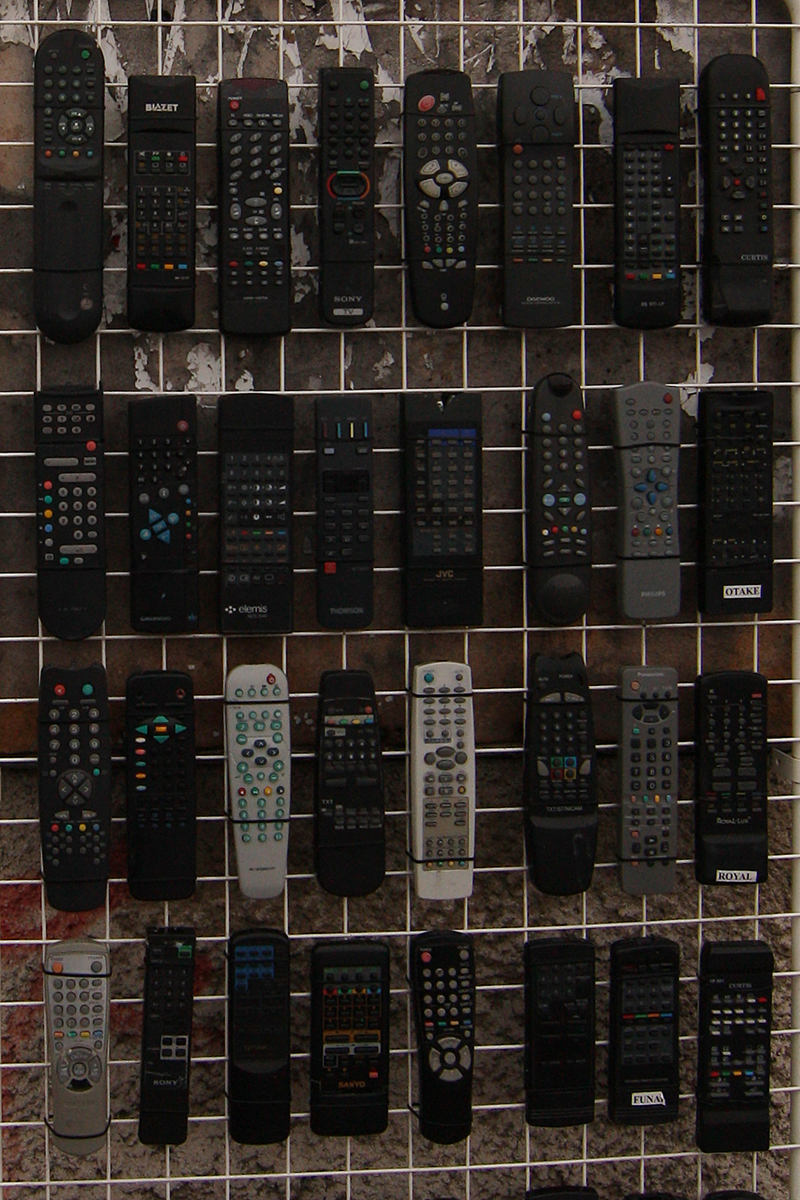The photograph features a display of remote controls meticulously arranged in a grid-like pattern against a marbled brick background, offering a striking visual contrast. The remotes are organized into four rows with eight units per row. The predominant color of the remotes is black, but there are also variations in gray and white, adding visual and functional diversity to the layout. The top row consists entirely of black remotes; the second row includes one dark gray amid the black ones; the third row introduces a light gray and a white remote; and the fourth row features a silvery gray remote alongside the black ones. Each remote varies in design, with differing button configurations, including some with red buttons and others featuring four colored buttons. They are all mounted on a wired rack, which appears to be white or gray. The setting suggests a flea market or store display, with the wired rack securely holding the assortment of remote controls against the varying shades of the brick background.